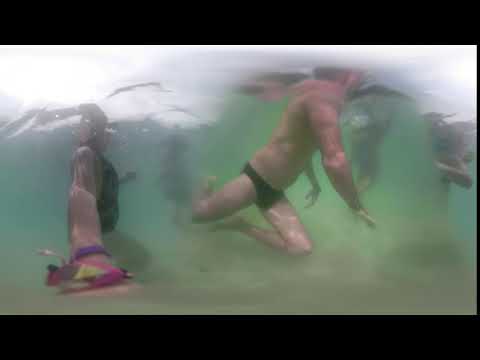The underwater scene captures a vibrant yet serene moment with several swimmers immersed in green-tinged water. At the center of the rectangular image, a man in a black Speedo commands attention with his arms extended forward and legs bent behind him, swimming gracefully. Surrounding him, other figures blur into the background due to the water's distortion, with one person identifiable by pink fins on the left. Vertical and horizontal black bars frame the top and bottom of the image, perhaps indicative of a window or underwater structure. The water's surface has a reflective white quality, mirroring the cloudy sky above, indicating the photo was taken outdoors possibly around midday. Although submerged, the scene is bathed in natural light, enhancing the varied colors: shades of black, green, purple, pink, and tan. The overall scene evokes a tranquil underwater escapade.